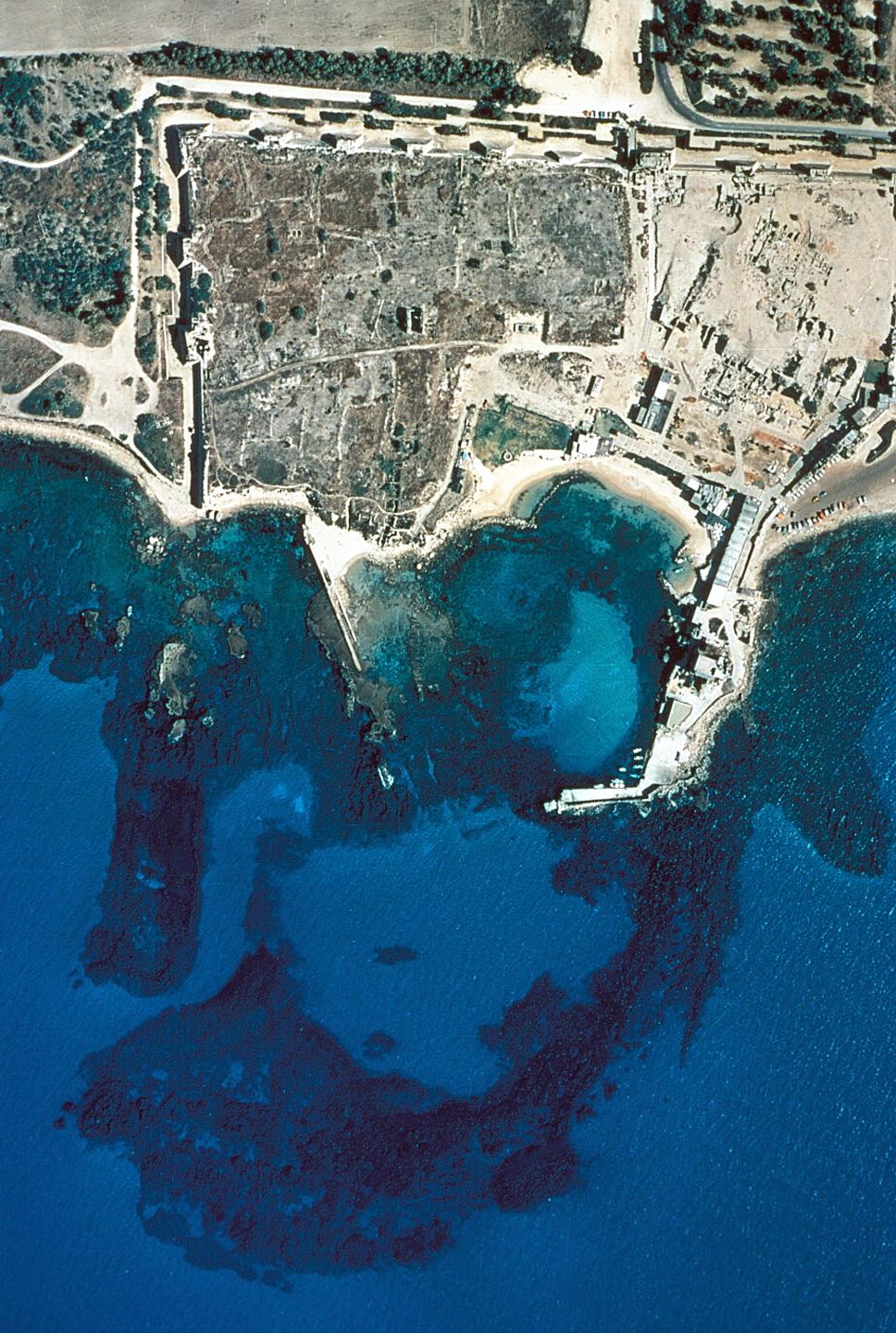The image is a color photograph captured from a high vantage point, possibly a satellite or plane, offering a sprawling view of a coastal town. The dark blue ocean dominates the bottom of the image, with hints of underwater land formations visible beneath its surface, including what appears to be a coral reef or some other underwater structure. Moving toward the center, sandy land formations emerge, transitioning into a more urban setting characterized by gray and brown buildings. Major roads traverse the town, connecting various parts from one end to the other. Verdant trees and plantations frame the man-made structures, adding patches of green to the scene. Notably, a desolate, barren area devoid of vegetation occupies the top right corner, suggesting a possible mining activity. Additionally, structures such as bridges protrude into the water, although no vehicles, people, or animals are visible in the photograph. The entire scene is captured in daylight, highlighting the natural and urban elements of this coastal town.